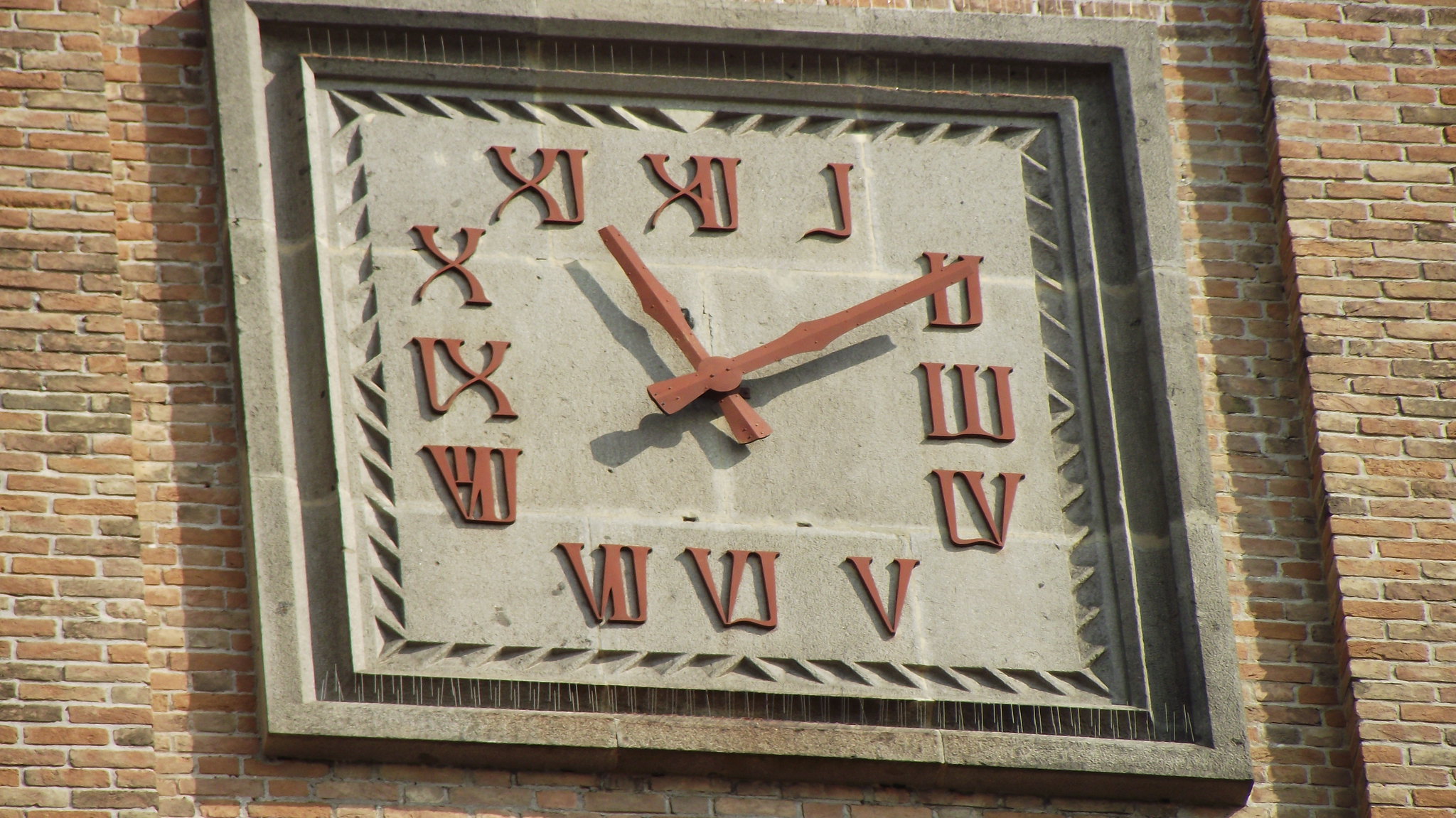The image depicts a square analog clock mounted on a brick wall, situated outside an unspecified building. The clock features a brownish-gray border and a tan-colored face, with light brown Roman numerals that are uniquely displayed in reverse, resembling a reflection. The time shown is 11:10, with no second hand present, only the minute and hour hands. The setting suggests it could be part of a diverse range of structures, possibly a school or a church, but its exact location remains a mystery.